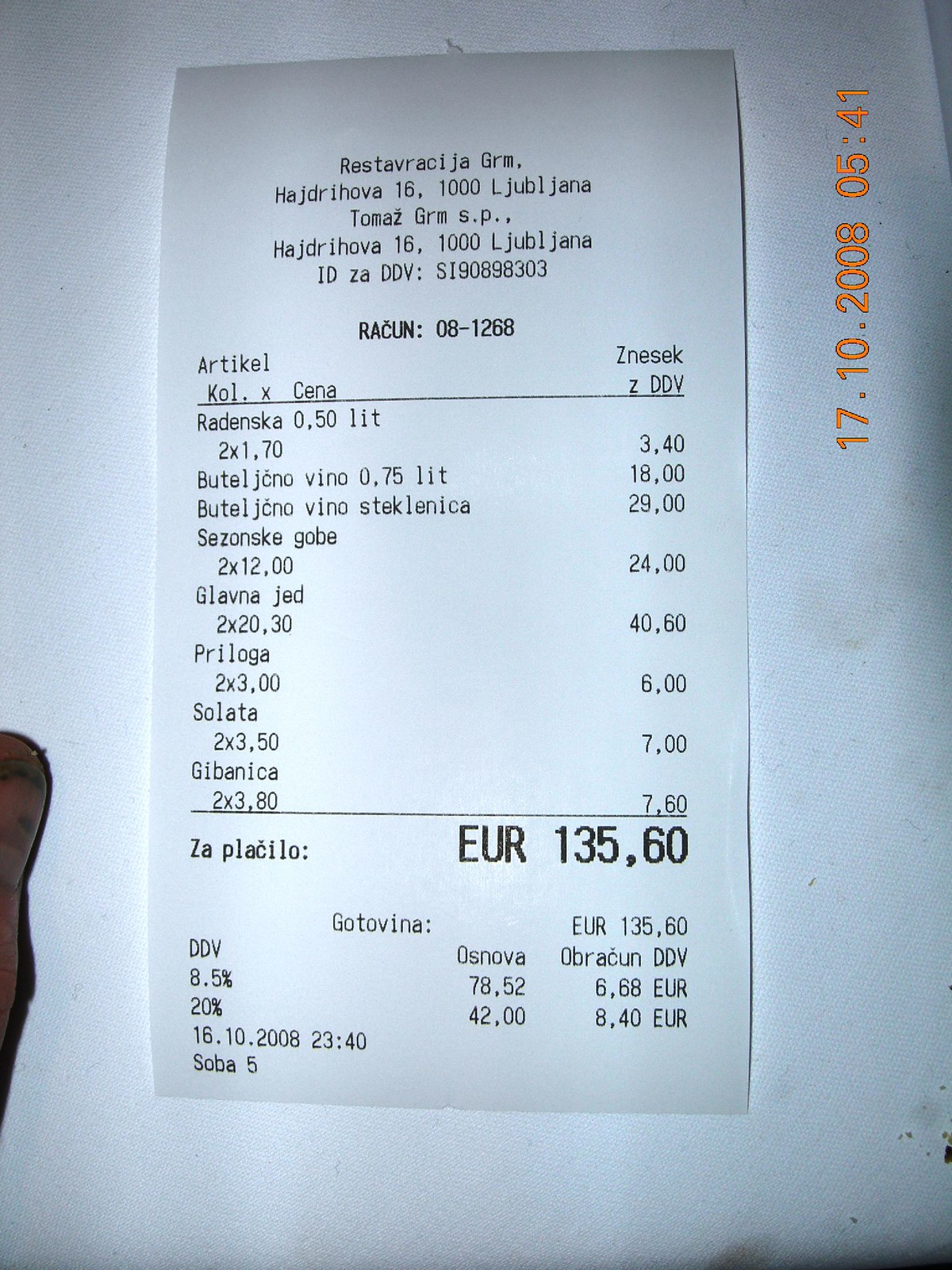This photograph captures a detailed close-up of a receipt placed on a white surface that might be a napkin or a paper towel, resting on what appears to be a table. To the left of the receipt, there is a partially visible object that could potentially be a person's hand or finger, indicated by a noticeable fingernail and a brownish hue. The receipt is printed in a language other than English and lists prices in euros. The total amount for the items on the receipt is 135.60 euros. Eight distinct items are detailed on the receipt. The header indicates the receipt is from a business located in Hadrihova, Ljubljana. Percentages listed on the receipt likely specify the taxes applied to the purchases.